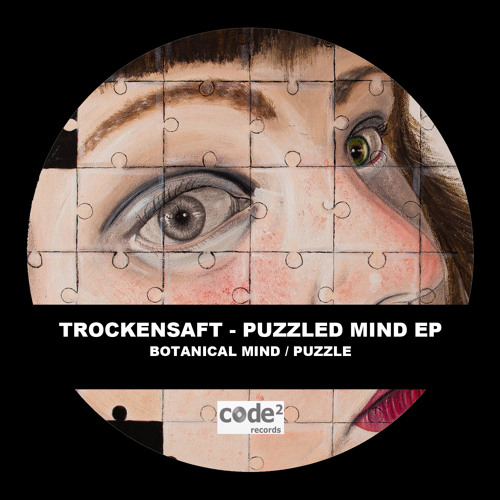The image presents a circular puzzle with a dark black background, depicting the illustrated face of a fair-skinned woman. Her expression is one of wide-eyed inquisitiveness or perhaps shock. The woman has blue eyes, though some details suggest her pupils or retinas might differ in color, and she has brown hair and eyebrows. Her lips are painted a striking red. Notably, a couple of puzzle pieces are missing in both the upper left and bottom left corners of the image. A horizontal black bar beneath her nose contains white text that reads "Trocken Saft Puzzle Mind EP Botanical Mind / Puzzle," with "Code Squared Records" positioned below it. This stylized puzzle emulates an album cover, merging a minimalistic and somewhat enigmatic visual theme, underscored by subtle variations in the woman's complexion, such as light tan skin tones and areas of redness suggesting either a slight rash or blushing.